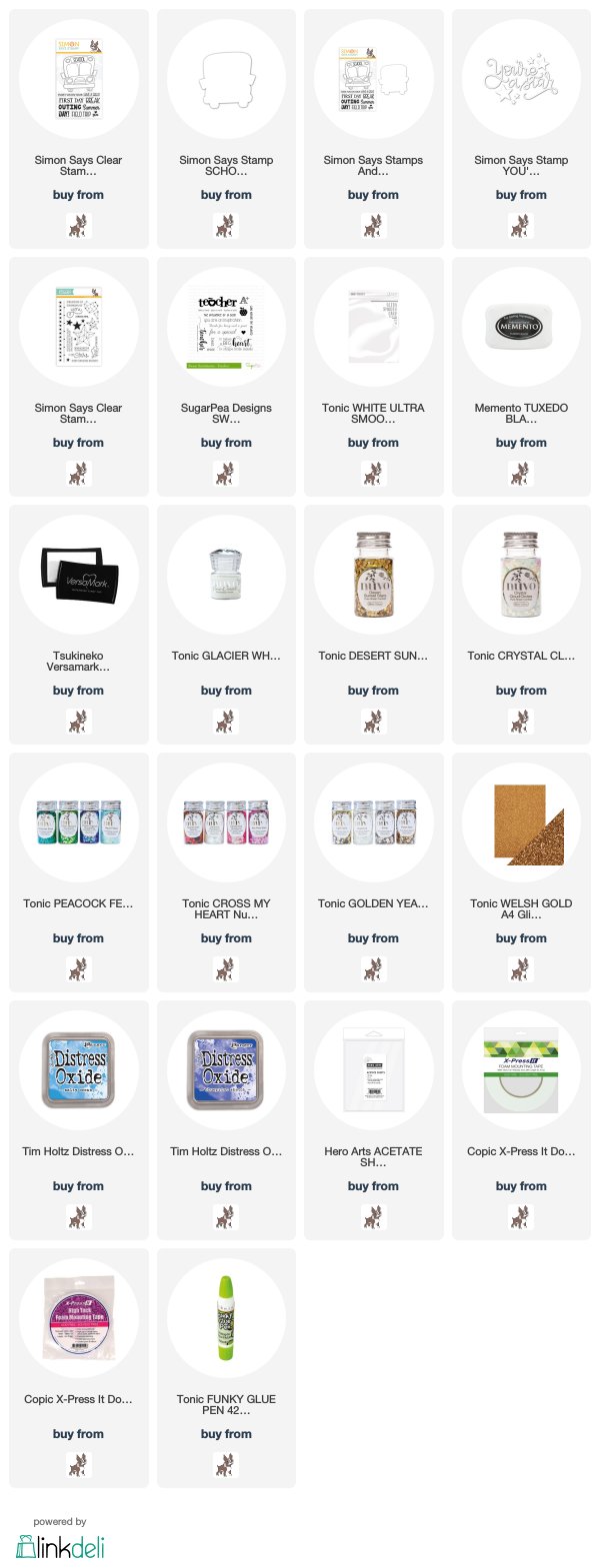The image features a total of 22 distinct tiles, each containing its own unique image. The tiles are arranged in a grid format and are uniformly designed with a background in very light gray. Central to each tile is an oval that houses a different image, making each tile visually distinct. Below each image, there's descriptive text in black, though this text is blurry and unreadable in the screenshot. Additionally, there is bolded black text in each tile, matching across all tiles, along with a small identical image accompanying this text. These consistent elements suggest some form of categorization or branding.

While the individual images on the tiles are unclear due to the screenshot's reduced size and resultant blurriness, they appear to represent products potentially from various countries, given their non-American appearance. The overall context implies a shopping or product browsing interface. The entire collection of tiles at the bottom of the screen is noted to be presented by Link Deli, suggesting a connection to the brand or platform facilitating this mosaic of images.